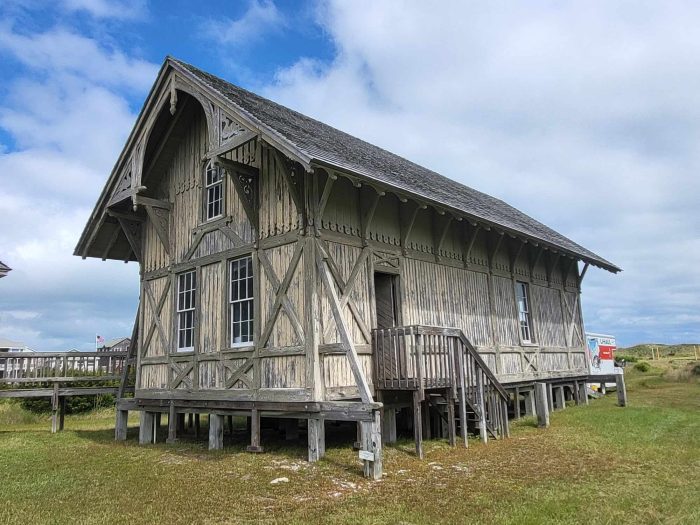The image captures a large, elevated wooden structure that resembles an old barn or church, possibly dating back 200 years, with elements that harken to historic architecture. The main building is constructed from grayish to light gray-brown weathered wood and is raised several feet off the ground on wooden stilts or columns, creating an open space beneath it. The structure is rectangular and elongated, featuring multiple windows on both the first and upper story. There is a small wooden staircase leading to a doorway on the front side.

The overcast sky dominates the upper portion of the photograph, filled with varying shades of light to dark gray clouds, with only a small patch of blue visible in the top left corner. A dark roof crowns the building, though only a sliver is visible due to the angle. Behind the structure, towards the center-right, a partially visible U-Haul truck is backed up to the building. The surrounding land is flat and grassy, interspersed with patches of dark brown soil where the grass is thin. In the distance, the American flag can be seen flying, further adding to the historical ambiance of the scene.